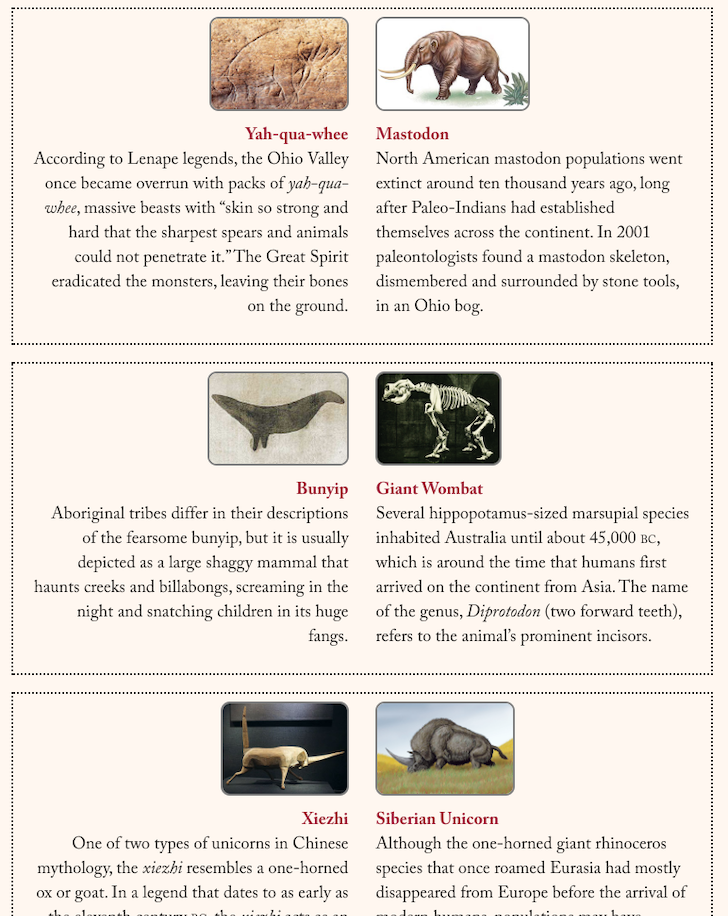The image is a detailed educational display resembling a textbook page, featuring six extinct or mythical creatures against a pinkish background, each with accompanying illustrations and descriptive text. At the top left is an etched stone carving labeled "Yaquawi," associated with Lenape legends describing armored beasts in the Ohio Valley. To its right is an illustration of a mastodon, noting their extinction over 10,000 years ago and a particular 2001 discovery in an Ohio bog. The middle row features the Bunyip on the left, depicted as a large, shaggy mammal from Aboriginal mythology, and the skeletal remains of a Giant Wombat with detailed information on its prehistoric existence in Australia, on the right. At the bottom left is the Chia Seed, a mythical one-horned animal from Chinese legends resembling an ox or goat, while the bottom right showcases the Siberian Unicorn, a prehistoric giant of Eurasia with a prominent horn that looks similar to a black bison.